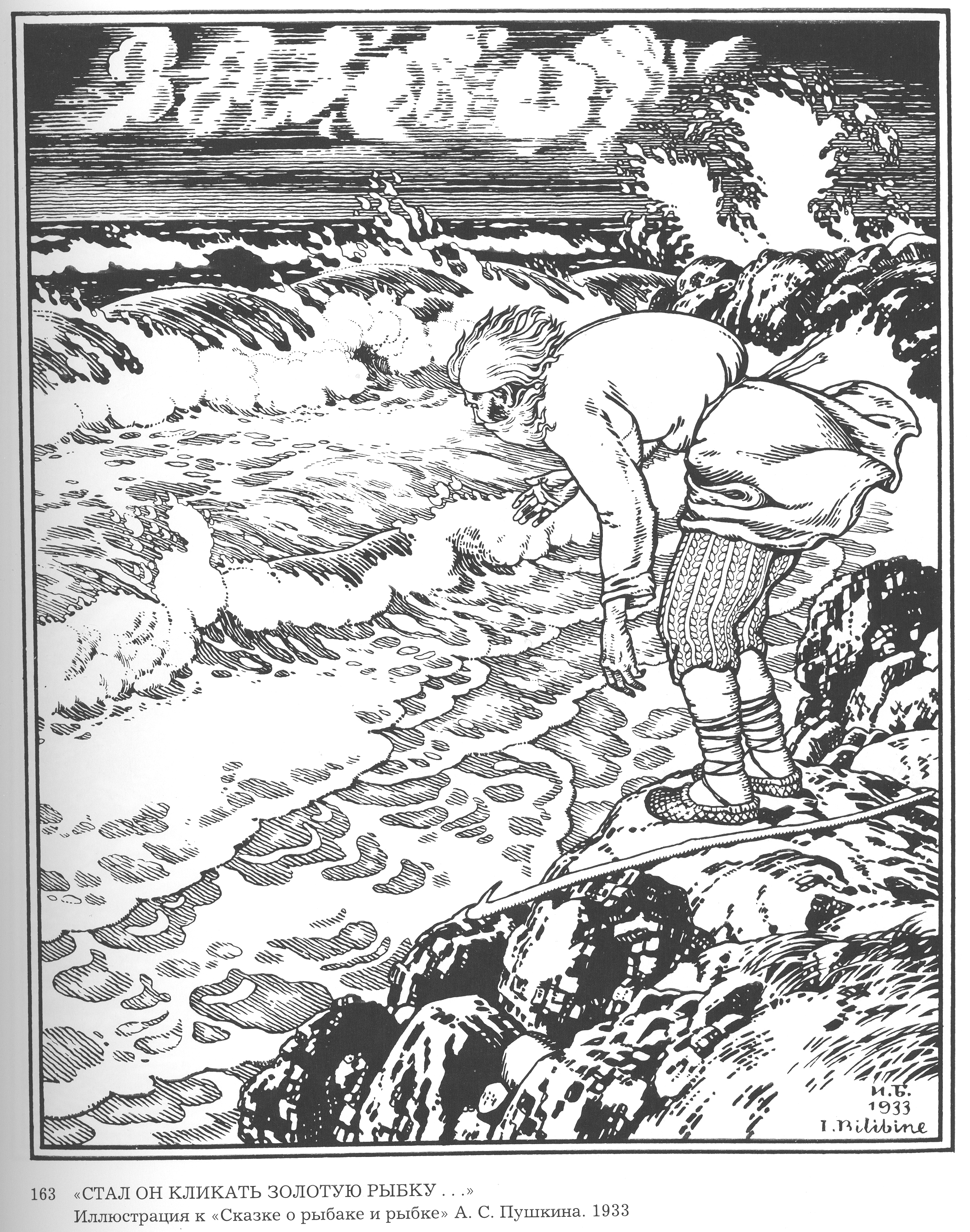In this detailed black-and-white sketch, an elderly man is depicted standing on rocky shorelines with violent waves crashing around him. The image is reminiscent of a comic book or woodcut style, marked by numerous precise lines. The man is portrayed with a flowing beard and long hair swept back by the wind, appearing in profile as he gazes down towards the turbulent sea. He is dressed in a tunic tied at the waist, wear short pants resembling cable knit, and sandals with laces extending up his legs. The scene is further dramatized by the menacing sea and clouds above, adding to the sense of impending action as he stands precariously close to the water. At his feet, a small stick lays on the rocks. In the bottom right corner of the image, there is text in another language, possibly Russian or Greek, which is not quite decipherable. The caption below this is signed "M.G. 1933" and includes the number 163, suggesting it might be an illustration from a historical publication.